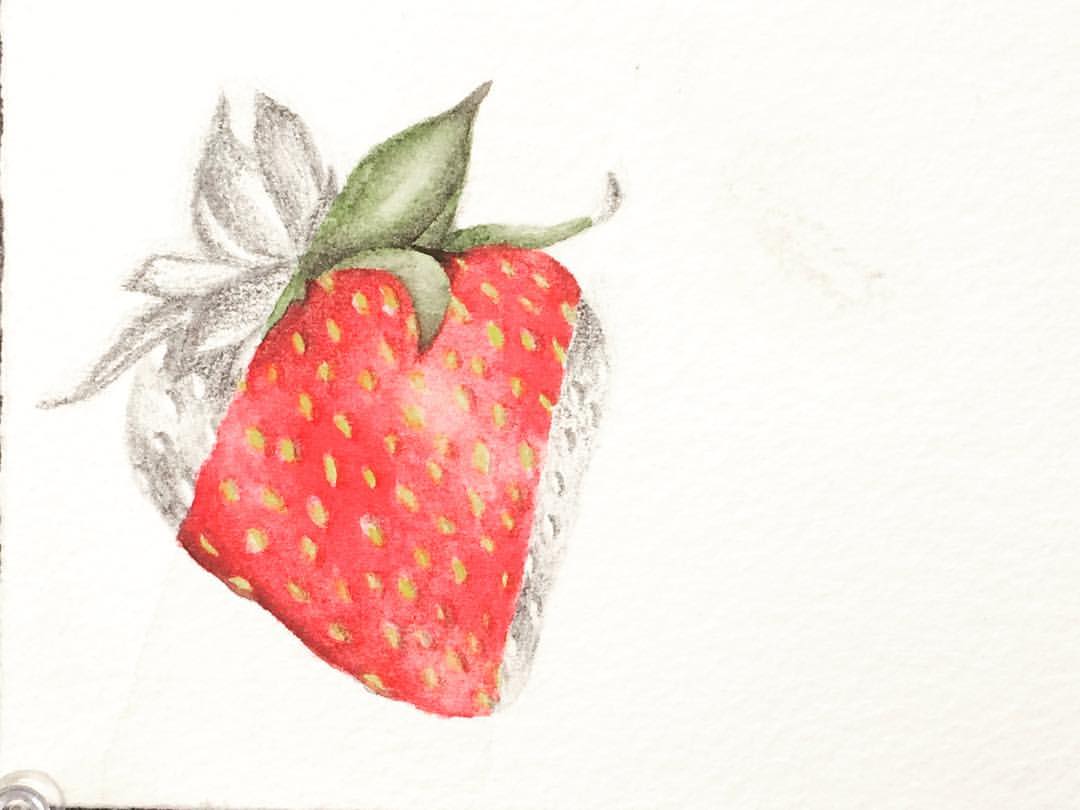This detailed close-up photograph features a hand-drawn illustration of a strawberry, rendered on a highly textured paper. The illustration combines both pencil and painted elements. The top left section of the strawberry, including portions of the leafy stems and part of the fruit's body, is depicted in pencil. Here, the rough pencil strokes interact with the textured paper, allowing white specks to peek through, adding a rustic charm to the image.

Contrasting this, the midsection of the strawberry is vibrantly painted, showcasing different shades of red that blend in a watercolor-like effect. The painted area also includes glossy, lighter sections to simulate the natural glare on the strawberry's surface. Scattered throughout this section are the characteristic yellow seeds of the strawberry, detailed with precision. Part of the green leafy stem is also painted, featuring dark green hues accentuated with white highlights, enhancing the leaf texture.

The remaining portion of the strawberry, rendered in pencil, mingles sketch-like quality with the textural richness of the paper. The interplay between the unfinished look of the pencil drawing and the vibrancy of the painted section creates an intriguing contrast, leaving the viewer to ponder whether the drawing is intentionally partial or yet to be completed.